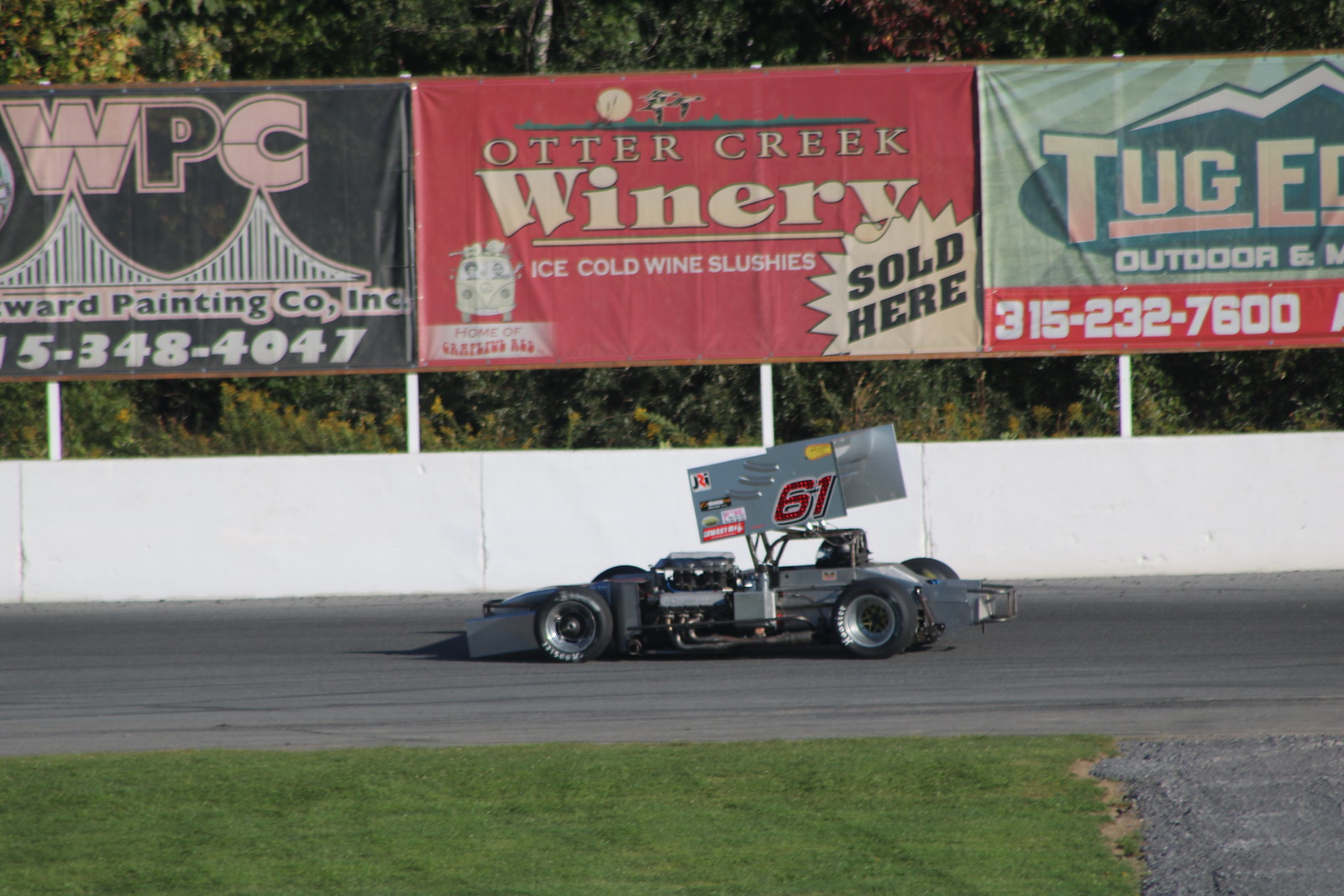This detailed image captures a race car at a racetrack, moving from the right to the left against a backdrop of assorted sponsor billboards. The silver race car, which is not part of the NASCAR or F1 series but resembles a winged sprint car, boasts distinctive features including large, fat tires, a roll bar, gray fins for track stability, and the red number 61 emblazoned on its side. The car races along the tarmac, bordered by a green grass infield and a white wall.

Rising above the fence are several colorful billboards. One advertisement is from WPC, Ward Painting Company, Inc., displaying the number 348-4047. Another billboard promotes Otter Creek Winery, highlighting their ice-cold wine slushies. Additionally, a partially visible sign mentions Tug Eco Outdoor with the phone number 315-232-7600. Beyond these advertisements, the scene is framed by a lush expanse of trees, completing the vivid and dynamic atmosphere of the racetrack.